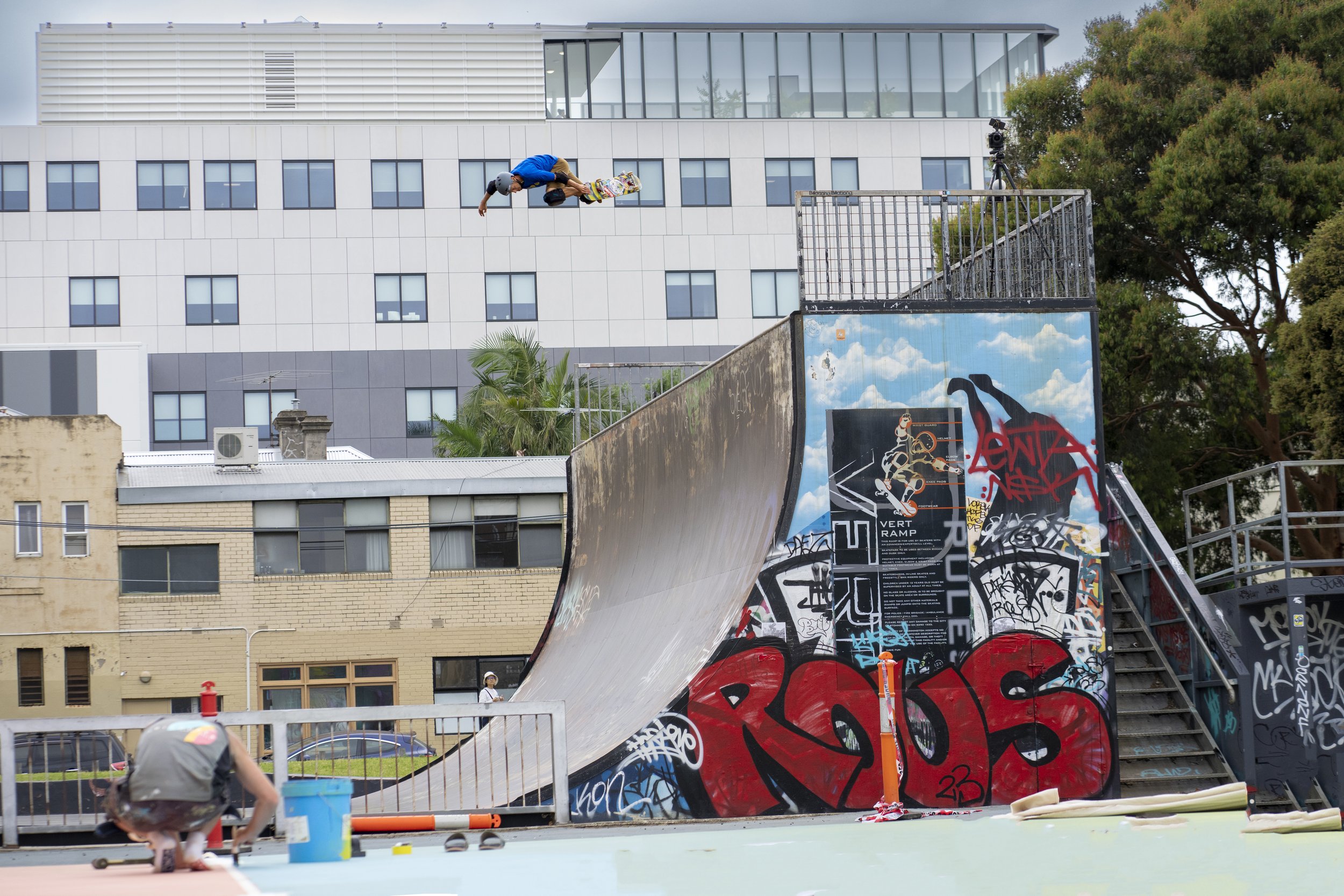In this vibrant outdoor scene, a skateboarder is captured mid-air, performing a trick on a large skate ramp. The skateboarder, dressed in a blue shirt, tan pants, gray helmet, and knee pads, is prominently featured against a backdrop of a blue sky dotted with white clouds. The ramp, likely a half pipe, is gray with a high, curved angle and heavily used white edges. It is decorated with colorful graffiti, including black, white, blue, and red markings, and features the text "R-O-U-S" in bright red at the bottom. 

To the right of the ramp, a gray staircase with silver railings leads up to the top, adjacent to a wall covered in white graffiti. A large, leafy green tree with brown branches stands in the upper right corner, providing a natural contrast to the urban elements. In the background, multiple buildings can be seen – a white building with many windows, especially at the top, and a gray-and-yellow building with gray and black framed windows and a glass panel with a black railing.

At the base of the ramp, a second skateboarder in a gray t-shirt and green pants is bending over next to a blue bucket with a white label. Nearby, two traffic cones, one tipped over and one upright, add to the scene's detail and color. The entire image is infused with bright, vivid colors, highlighting the dynamic energy of the skateboarding action and the surrounding environment.